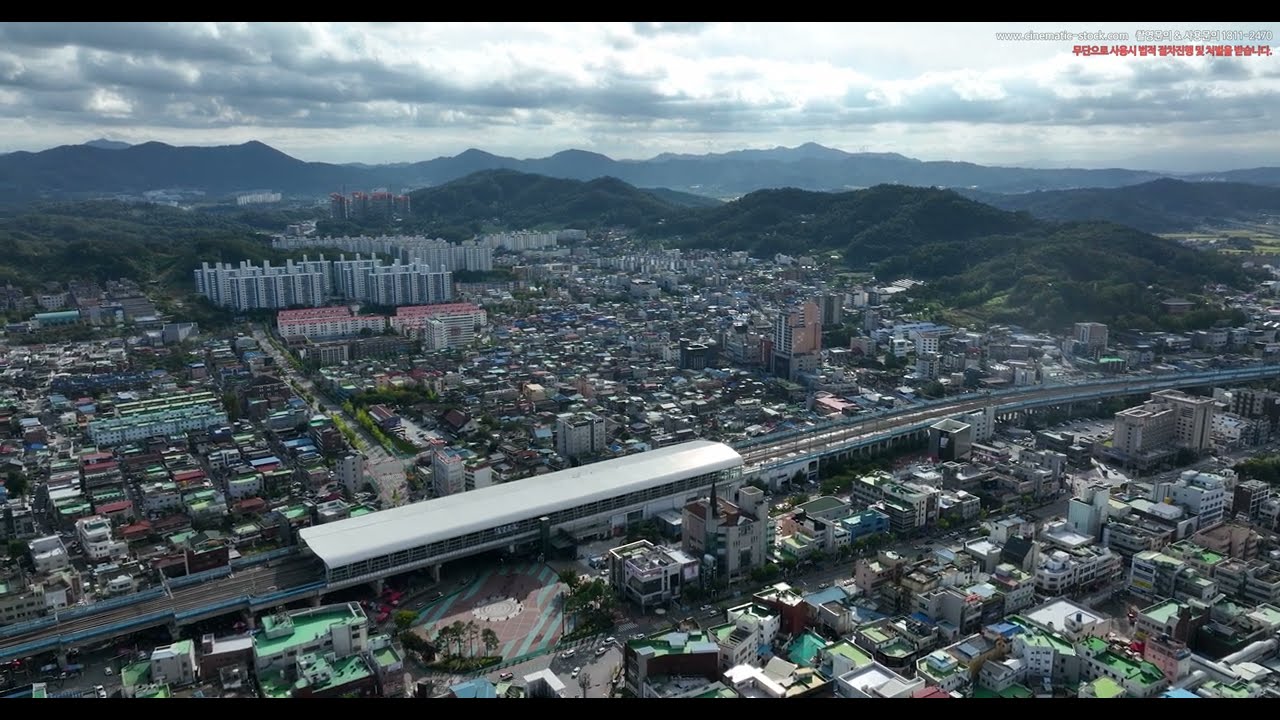An aerial view captures a large, dense city sprawling from the bottom left to the center of the image and extending towards the right. The city is marked by numerous intertwining roads and colorful buildings, including high-rise and apartment structures, converging into a dense, rectangular pattern. Slashing diagonally from the bottom left to the center right, a raised railway track stands out, featuring a covered silver platform or hub with a distinctive white roof and dark siding. This railway effectively bisects the city, adding a linear element to the urban sprawl.

Beyond the city's confines, grassy green hills transition into a range of darker gray mountains, forming a layered backdrop. These natural features surround and rise above the urban landscape, with the tallest peaks visible in the far distance. The sky above is filled with a blend of light and dark gray clouds, contributing to the overcast ambiance of the scene. The entire image is framed by thin black bands at the top and bottom, subtly enclosing the view. Additionally, textual elements in white and red Korean characters overlay the image, including the web address "www.cinematic-stock.com" and the numbers "1811-2470."